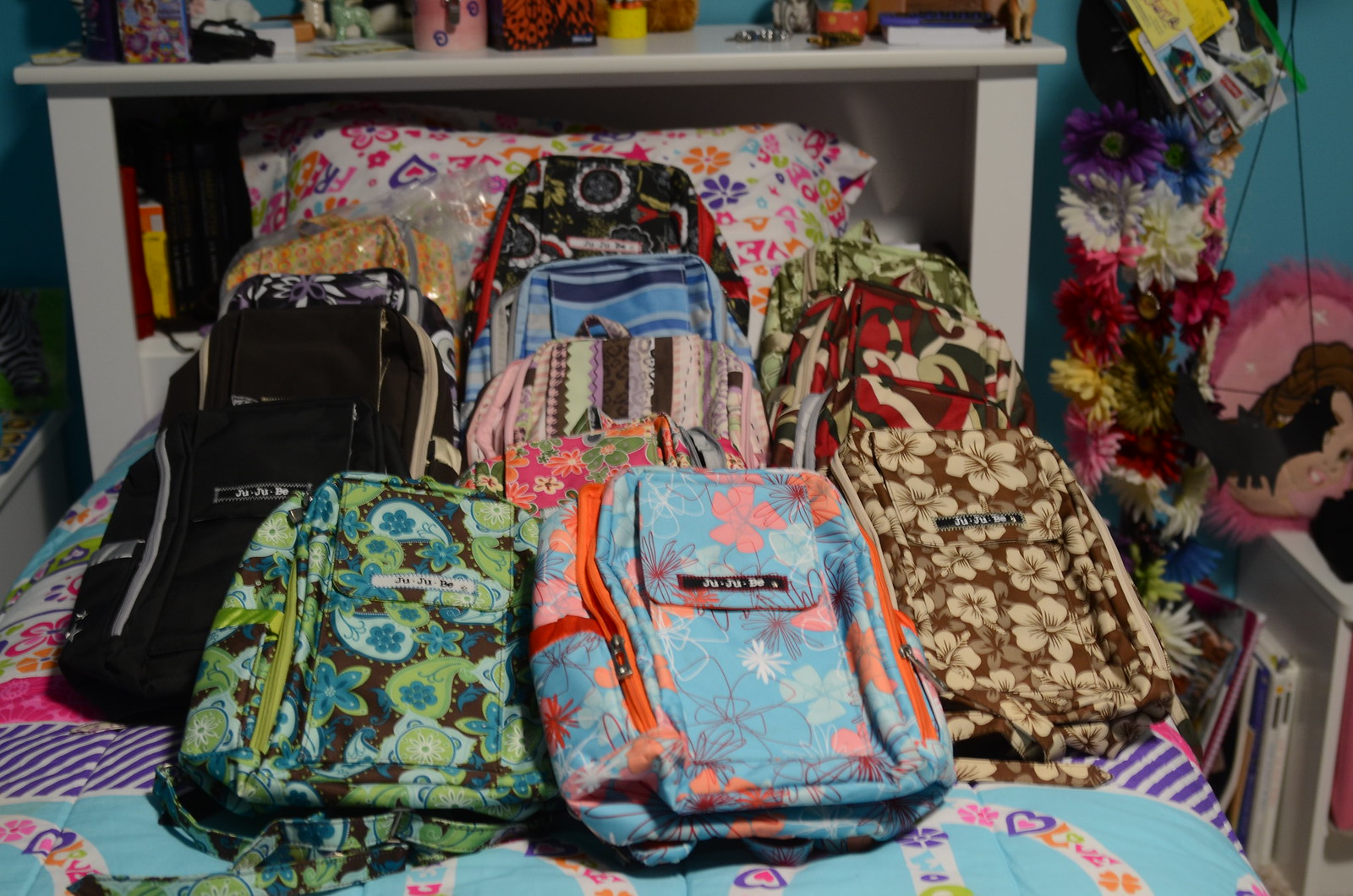In a vibrant children's room, a color photograph captures an array of backpacks meticulously arranged on a girly-themed bed. The bed is adorned with a lively, multicolored bedspread featuring patterns of hearts and flowers in various shades of blue, purple, pink, orange, and green. A white wooden bed frame doubles as a shelf, holding an assortment of knick-knacks and books. Draped beside the shelf, a floral lei adds a touch of whimsical charm. 

At the heart of the photograph, several backpacks—bearing the Jujube logo—occupy the bed's center, each showcasing unique prints and colors. The designs range from floral and paisley patterns to solid black and camouflage prints. Notable variations include a dark brown backpack with white flowers and accents, a light blue one with pink and blue floral patterns, and a greenish-blue one adorned with vibrant flowers. There are also solid black, striped, and colorful camouflage backpacks, each with distinct zipper colors. Behind the backpacks, a brightly colored pillow with matching heart and flower motifs complements the pastel-colored bedding. The arrangement of bags suggests they might be presented for sale, carefully overlapping one another in a visually appealing display.